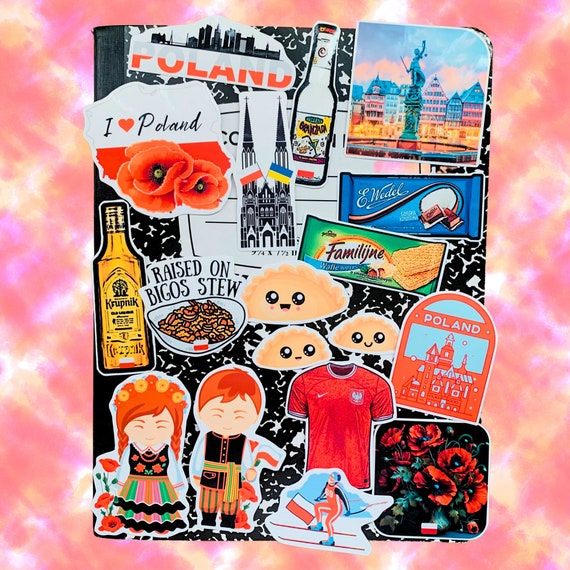The image features a vibrant tie-dye or psychedelic background in bright pink and yellow hues. In the center, there is an open black-and-white composition booklet, the kind with black binding and marbled print on the cover, labeled as a composition book. The cover is adorned with various stickers, all with a Polish theme. 

One prominent sticker says "Poland" with the top halves of the letters in white and the bottom halves in red, featuring a large city. Another sticker depicts the Statue of Liberty, while yet another reads "I love Poland" or "I heart Poland" with coral-colored poppies beneath the word Poland. Among the stickers, there is one that states "raised on Big O's stew" in black text, and there are red flowers scattered around.

Additional stickers include an orange one at the top and images depicting Polish towns, a church with two towers, and a Polish and Ukrainian flag together. There are also stickers of bottles of alcohol, a Nike shirt with an eagle design, and one showing a red jersey with a white Nike swoosh and a lip mark. Other stickers feature traditional Polish scenes, such as a girl skiing, a man and woman in traditional Polish costumes, and depictions of traditional foods like pierogies.

The collection of stickers, including Polish flags (white on top, red on the bottom), creates a collage that celebrates Polish culture and heritage within the whimsical background.